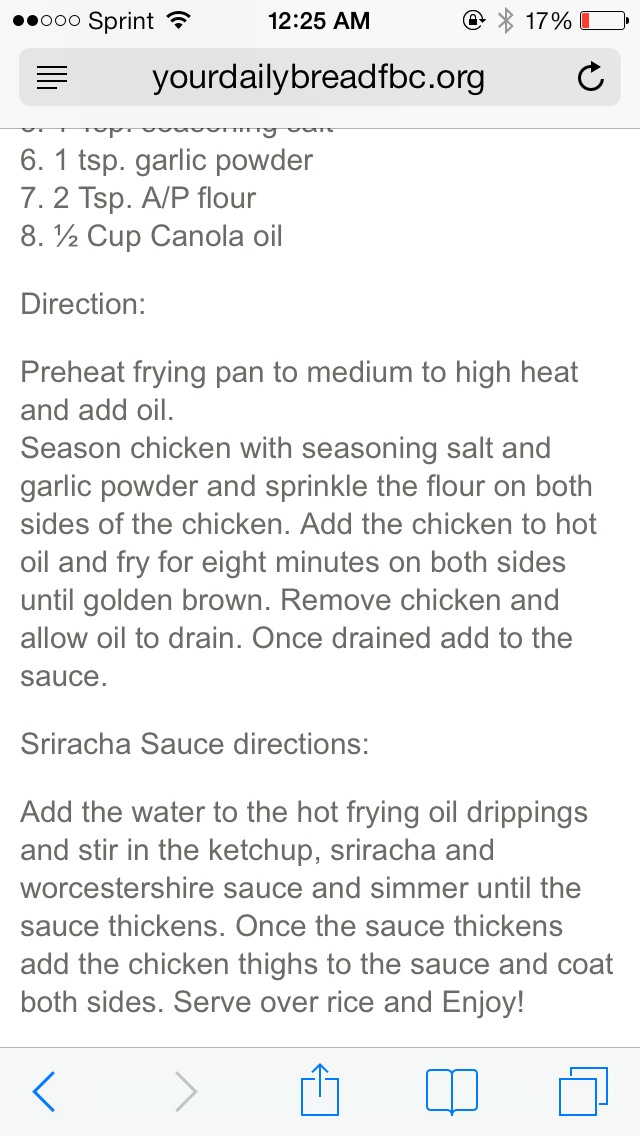The image is a screenshot of a recipe displayed on a smartphone, with details revealing it was accessed on a Sprint network at 12:25 a.m. The phone's battery is at 17%, indicated by a red sliver in the battery icon, urging a charge. The recipe is hosted on the website yourdailybreadfbc.org, visible below the interface elements which include signal strength bars and connectivity icons. The recipe details the final steps needed to prepare a dish, focusing on seasoning and frying chicken thighs. Instructions include preheating a frying pan over medium-high heat, adding canola oil, and seasoning the chicken with seasoning salt and garlic powder. The chicken is then coated with all-purpose flour, fried in hot oil for eight minutes on each side until golden brown, and set aside to drain. The directions continue with the preparation of a sriracha sauce: adding water to the oil drippings, stirring in ketchup, sriracha, and Worcestershire sauce, and simmering until the sauce thickens. Finally, the fried chicken is coated in the thickened sauce and served over rice. The browser interface at the bottom of the image features navigation icons, including arrows and a sharing symbol, integral to smartphone use.